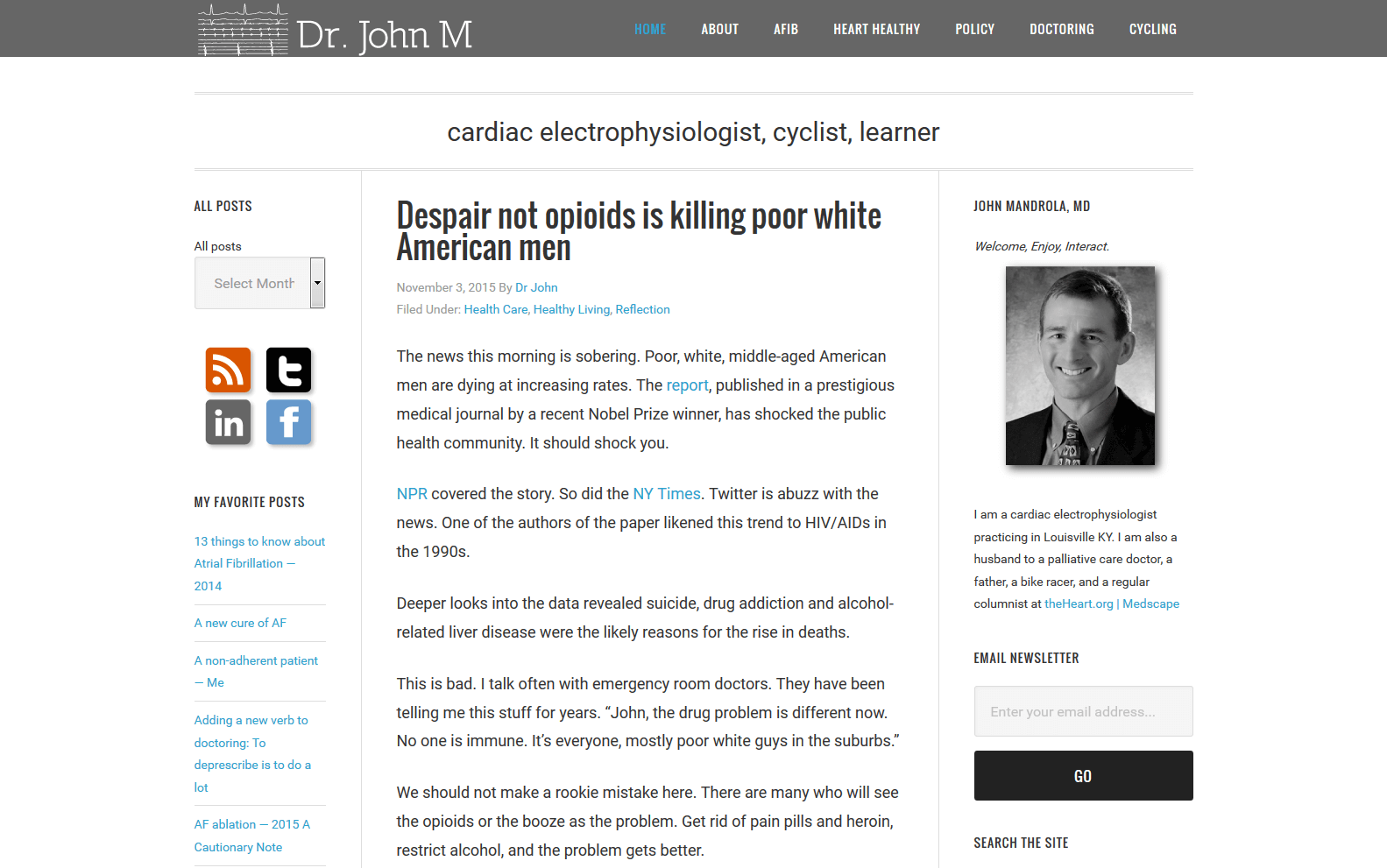Dr. John Lovell, a renowned cardiac electrophysiologist, avid cyclist, and lifelong learner, is featured in this detailed image. To the left of his black-and-white portrait, there is a series of social media icons: an orange square with a Wi-Fi symbol, a black square with a white "T," a gray square with the letters "IN" in white, and a blue square with a white "F." Dr. Lovell is depicted in the photograph dressed in a smart black suit, complemented by a dark dress shirt and a black tie, exuding professionalism and dedication. Below the portrait, there is an article titled "Despair Not: Opioids are Killing Poor White American Men," exploring the devastating opioid crisis.